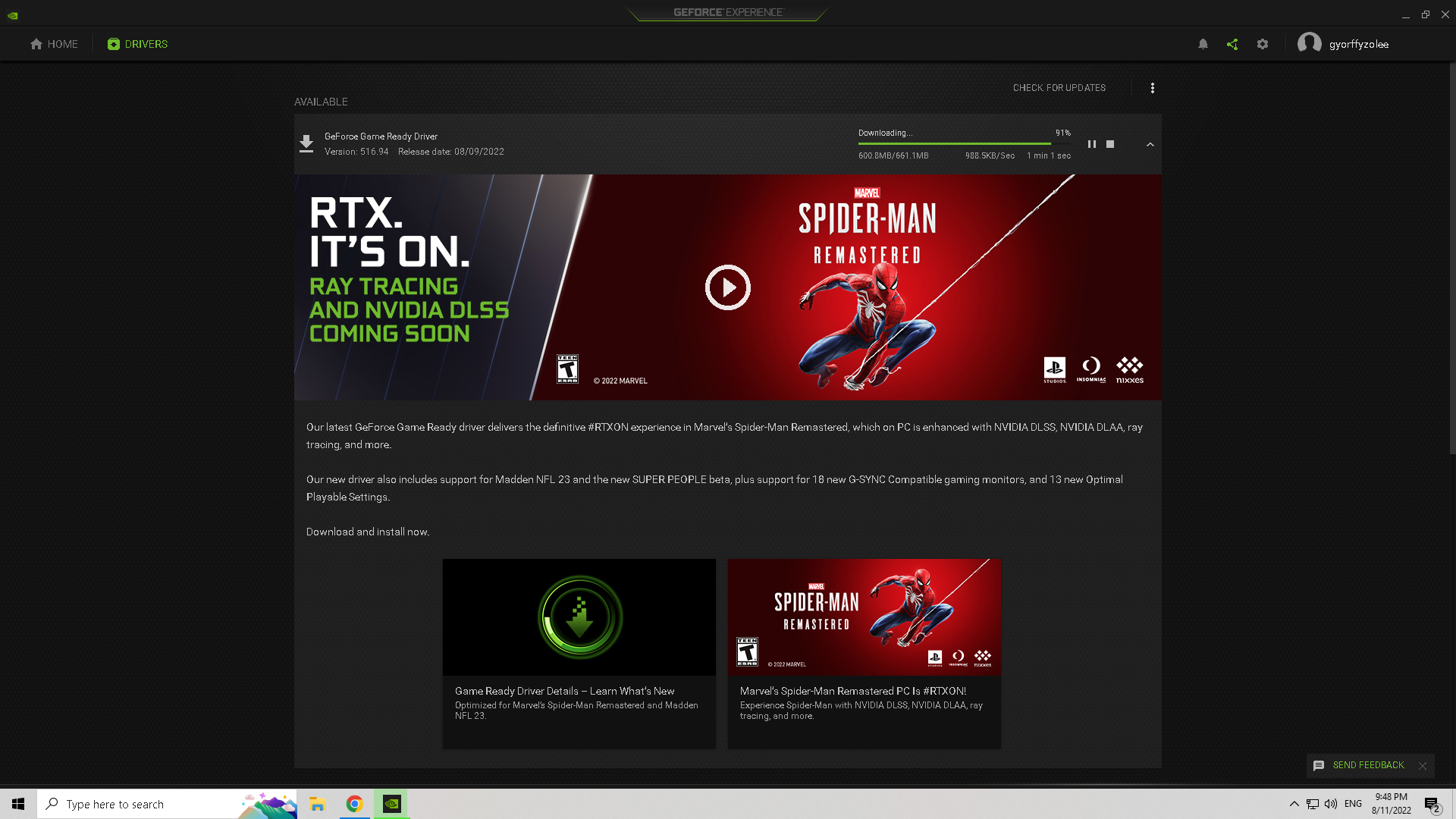This image is a detailed screenshot of the NVIDIA GeForce Experience interface during an update for the GeForce GameReady driver, version 516.94, released on August 9, 2022. The update progress is prominently displayed, with the download currently at 91%. The interface provides real-time statistics such as download speed in megabytes per second and the estimated time remaining for the download to complete.

The screenshot also showcases the user's profile in the upper-right corner, with the username "GYORFFYZALEE" clearly visible. An advertisement for "Spider-Man Remastered" is featured, displaying a play button likely intended to launch the game trailer. The main interface uses a sleek black theme, with a navigation bar at the top left containing 'Home' and 'Drivers' tabs, the latter highlighted in green to indicate the current page.

Additional interface elements include share and settings icons located to the right of the navigation tabs, providing quick access to those functions. The overall layout and design typify the user-friendly and immersive experience characteristic of the NVIDIA GeForce Experience software.